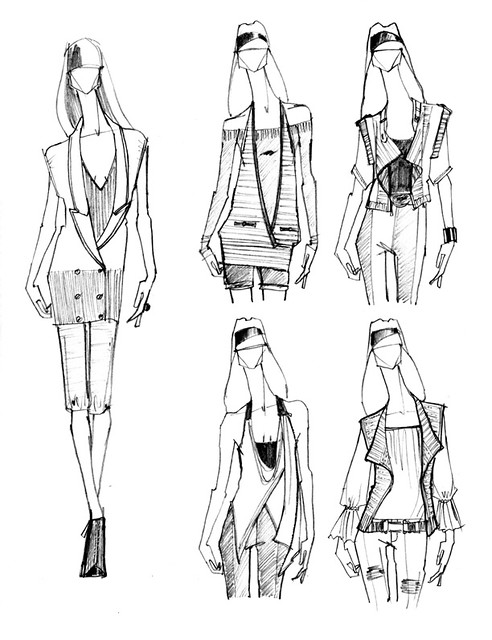The image is a fashion concept sketch on a white background, showcasing five female figures in black and white. The leftmost figure occupies about one-third of the image and is a full-body illustration of a faceless, tall model with elongated proportions, especially noticeable in the neck area. She has long hair with bangs and wears an oversized blazer as a dress paired with short capris, complemented by a black headband or bandana. The remaining four figures, which take up the other two-thirds of the image, are drawn from the thighs up, each depicting different outfits. These outfits include a variety of flowy, baggy styles, and amongst them is a short leather jacket paired with pants. Each outfit represents distinct, conceptual fashion designs, maintaining a consistent style across all illustrations.